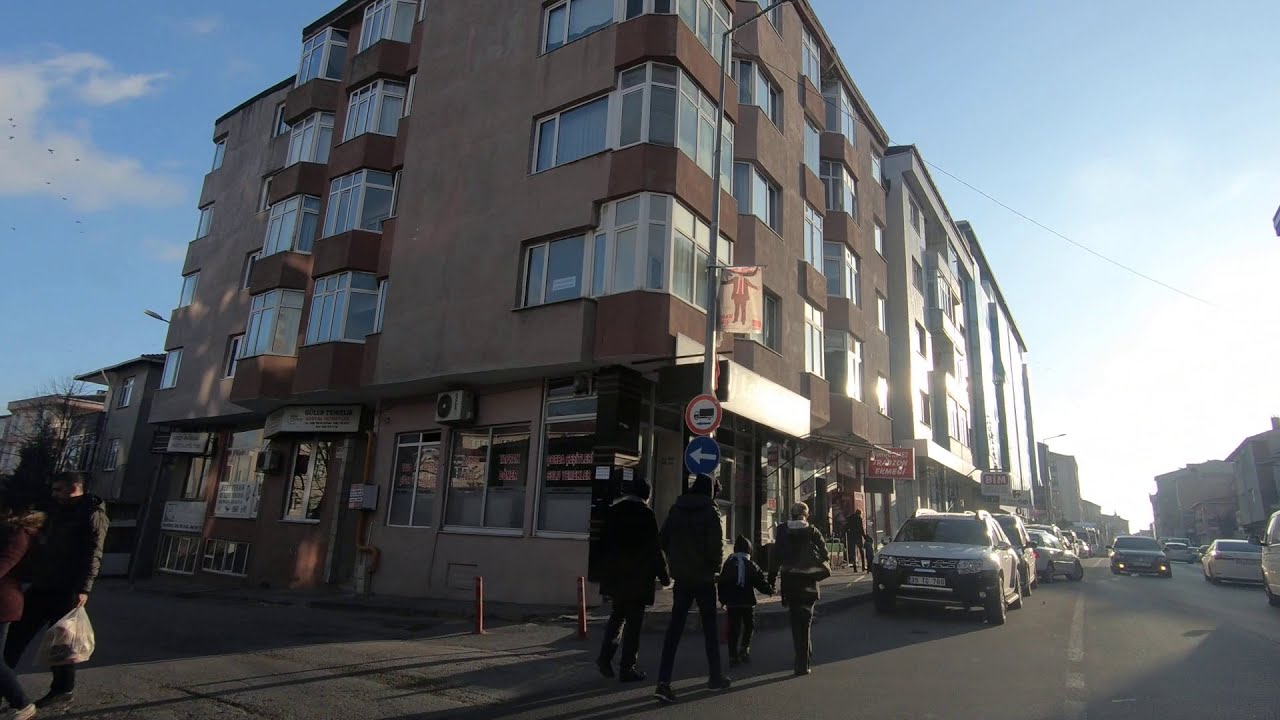This high-contrast photograph captures a lively urban street corner bathed in sunlight. The focal point is a rectangular building with a shop on the ground floor, indicated by signs and advertisements on a light pole in front. Above, four floors of windows suggest residential apartments. The architecture is sleek, devoid of balconies. On the right side, cars, primarily coupes, are parked with a black car driving toward the viewer, its bottom yellow circle lights on. People are walking around the bottom left, including a man dressed in black with a white sack in his left hand. At the center, a family of four consists of two men, a mom with dirty blonde hair, and a child in a black beanie; they all appear to be dressed in black. The sky is blue with scattered clouds, and the bright sun highlights the busy street, enhancing the bustling ambiance.